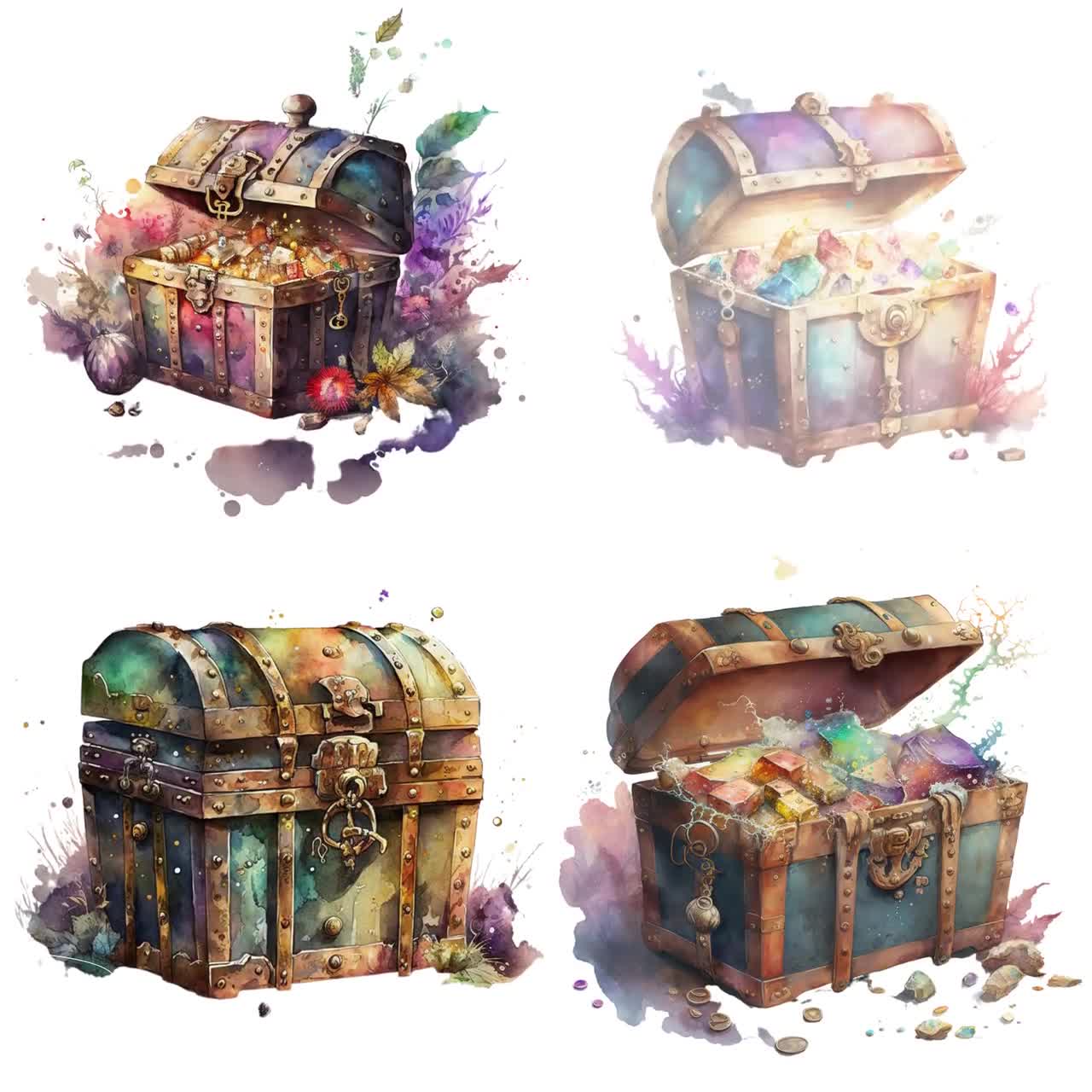The image features a collection of four detailed, digitally illustrated treasure chests arranged in a 2x2 grid. Each chest shares a similar shape with greenish hues and brass or gold straps. They are adorned with large central locks and surrounded by splotches of dark watercolor paint.

1. The upper left chest is partially open and angled slightly to the left. It showcases a burst of color inside, suggesting a treasure within, although specifics are hard to determine. A red fruit, a skeletal figure, and a plethora of bright hues, including yellow, purple, and blue, surround the chest. Additionally, leaves and a flower peek out from the right side.
  
2. The upper right chest is painted in faded purple and pink tones and is three-quarters open. Though its contents are somewhat ambiguous, it appears to be filled with bright treasures, possibly gems, all under a translucent filter. Surrounding this chest are pink and purple plants, enhancing its ethereal appearance.

3. The lower left chest is firmly shut and locked, displaying a combination of orange, blue, and green accents against its brownish body. It has a darker tone compared to the others, and watercolor splotches are visible to its left and right sides.

4. The lower right chest is three-quarters open and showcases a mixture of vibrant colors inside, hinting at various treasures. This chest is equally lively, with splotches of purple, yellow, red, and green, and is circumferenced by stones and darker watercolor splashes on the encompassing ground.

In summary, the image captivates with its collection of four vividly illustrated chests, each brimming with color and enigma, embedded in a setting of dark watercolor artistry.